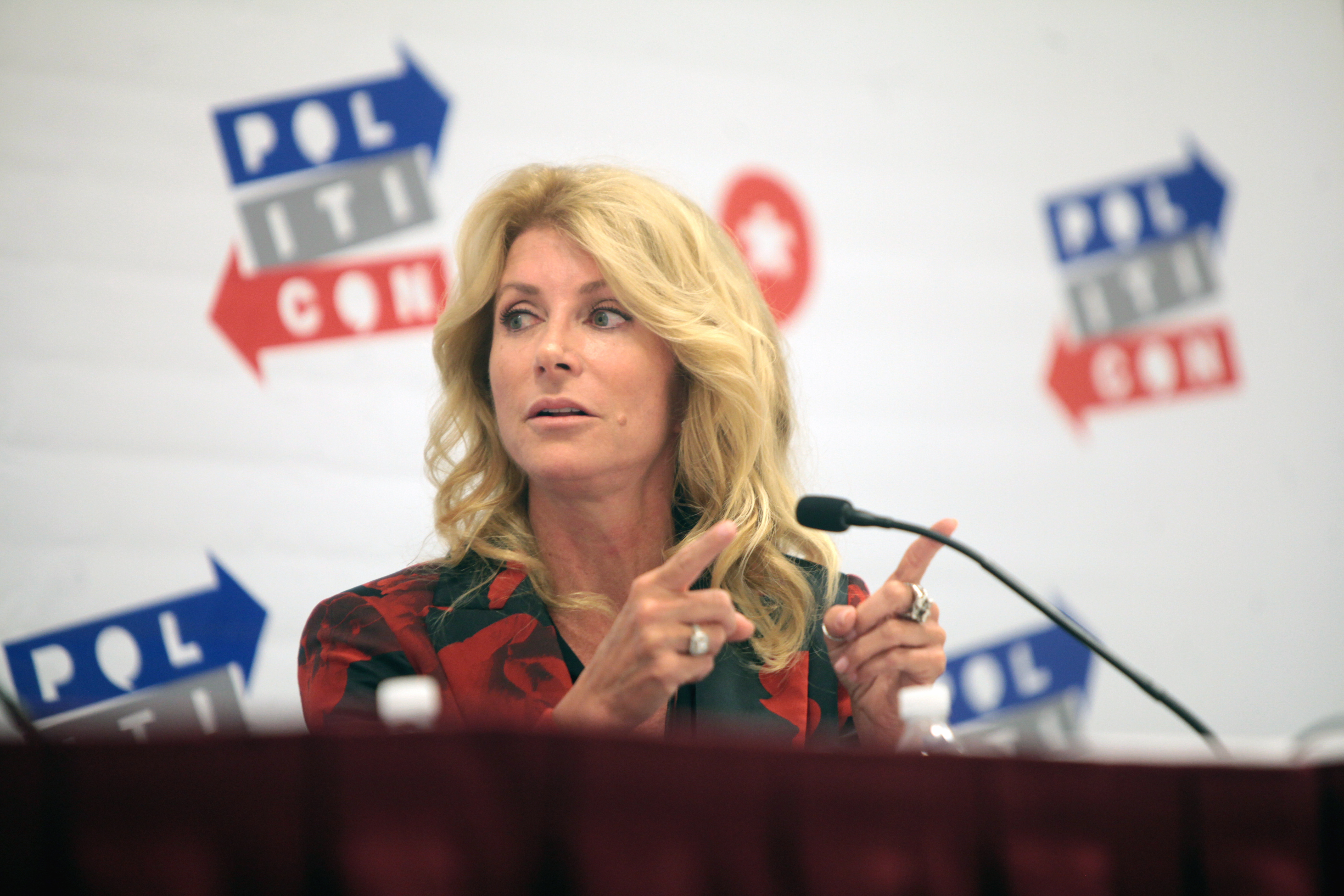The image captures a middle-aged Caucasian woman with long, wavy blonde hair cascading past her shoulders. She is seated behind a wooden desk, adorned with a microphone on a thin black stand positioned to her right. The woman is engaged, mid-dialogue, her mouth slightly open, and her head turned to the left while her body faces forward. She is dressed in a black blazer with red rose patterns and a black collared shirt beneath it, exemplifying business attire. The woman sports a wedding ring on one hand and a silver ring on the index finger of the other, both hands raised with index fingers pointing to the top right of the image. The background is a white banner repeatedly featuring the "Politicon" logo, composed of a blue arrow, grey box, and a red arrow, indicating her participation in a conference or political event. The intricate details of her attire and the dynamism of her gesture lend a compelling and authoritative presence to the photograph.